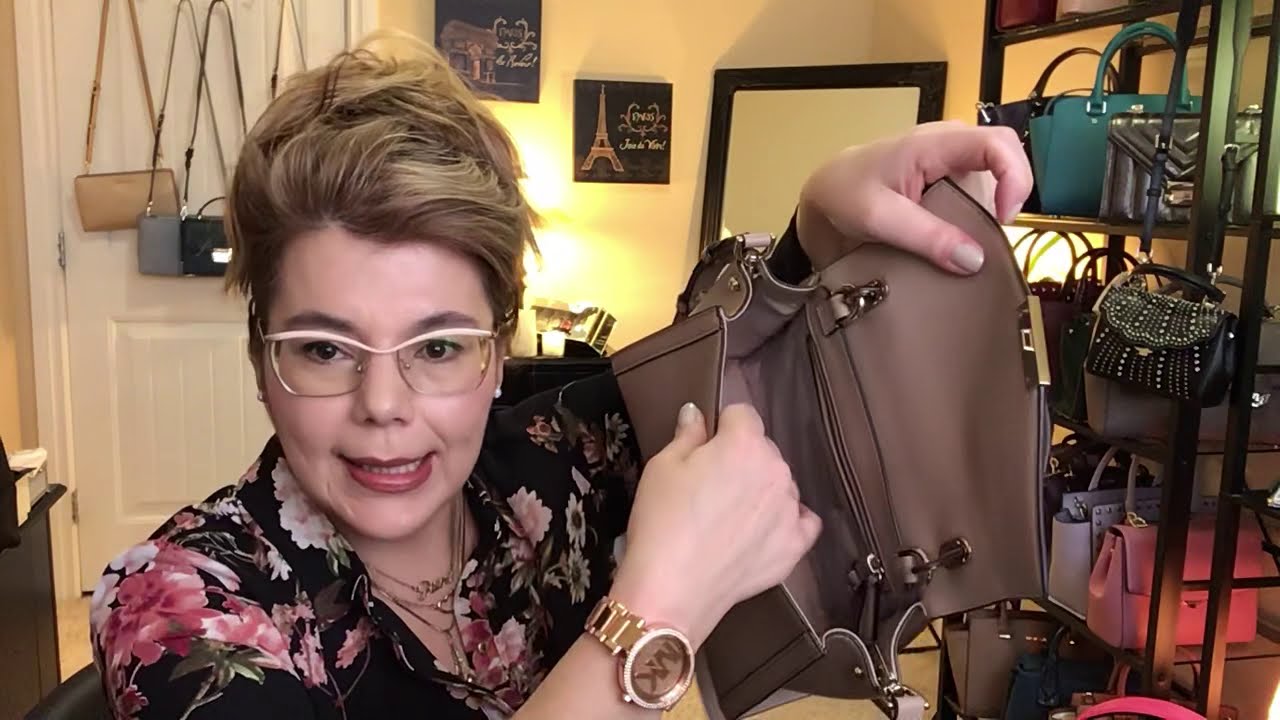In the image, a Caucasian woman with short blonde hair styled in an updo is presenting a tan brown handbag, showing its interior. She is dressed in a black blouse adorned with pink and white floral patterns and wears golden-framed glasses with a white stripe on top. A golden MK watch shines on her wrist. The setting is a spacious room filled with various handbags. Behind her is a white wall with numerous handbags hanging on it, and to her left is a closed white door also decorated with hanging purses. To the right, a light yellow wall displays two black and gold artworks, adjacent to a mirror with a black border. A black shelving unit on the right-hand side of the image holds an assortment of handbags, including pink, brown, aqua green, and some embellished with white rhinestones.